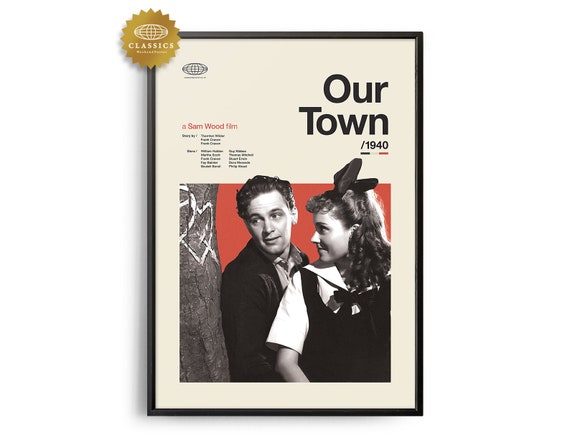The image is a poster print for the classic movie "Our Town," released in 1940. The print is encased in a black picture frame and displayed against a blank wall. The background of the print is a solid cream color. At the top left of the poster, there is a small globe, with an emblem above it that reads "Classics," resembling a gold medallion. 

To the right, in very large black font, is the title "Our Town," followed by the year "1940." Directly beneath the year, there are three very thin bars: blue, white, and red from left to right. To the left of the poster, the text "A Sam Wood Film" appears in red font, and beneath it is a list of words in black font that are too small to read, likely credits or a cast list.

Dominating the lower half of the poster is a black-and-white photograph of two young characters, set against a red background that appears to have been added digitally. To the left of the characters stands a brown tree trunk, with a heart and an arrow carved into it in white. The man, dressed in a black jacket over a gray shirt, leans his right arm against the tree, with brown hair and a contemplative look cast to the side. The woman, dressed in a black dress with a white sailor-collar shirt and a black bow at the neckline, has light brown hair styled with an oversized black bow that resembles animal ears. She stands with her back to the man, looking over her shoulder at him. The captured moment exudes a timeless, nostalgic charm reflective of the film's era.